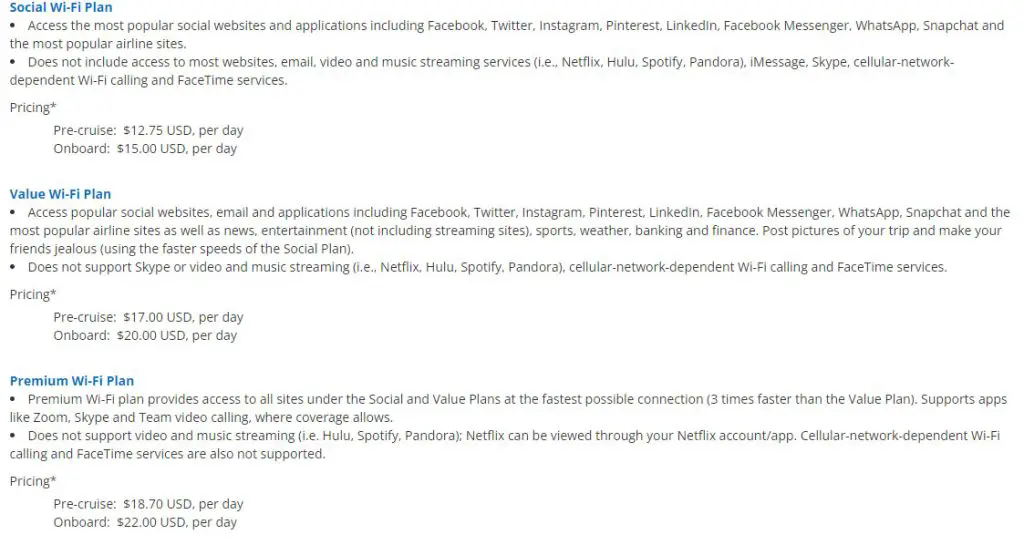This image is a screenshot from an unidentified website displaying three different Wi-Fi plans available for purchase. Each plan is organized into a distinct section with the titles highlighted in blue text, while the descriptions are in black.

1. **Social Wi-Fi Plan**: This plan allows access to popular social websites and applications such as Facebook, Twitter, Instagram, Pinterest, LinkedIn, Facebook Messenger, WhatsApp, and Snapchat, along with the most frequented airline websites. However, it does not support access to most other websites, email, or video and music streaming services like Netflix, Hulu, Spotify, Pandora, nor does it support iMessage, Skype, cellular network-dependent Wi-Fi calling, and FaceTime services. The cost is $12.75 per day if purchased before the cruise and $15 per day if purchased onboard.

2. **Value Wi-Fi Plan**: The Value Wi-Fi Plan grants access to popular social websites, email, applications including Facebook, Twitter, Instagram, Pinterest, LinkedIn, Facebook Messenger, WhatsApp, Snapchat, and leading airline sites. It also covers news, entertainment (excluding streaming sites), sports, weather, banking, and finance websites. Users can share photos from their trip and enjoy faster speeds compared to the Social Wi-Fi Plan. This plan does not support Skype, video and music streaming services like Netflix, Hulu, Spotify, Pandora, or cellular network-dependent Wi-Fi calling and FaceTime services. Pricing is set at $17 per day pre-cruise and $20 per day onboard.

3. **Premium Wi-Fi Plan**: The Premium Wi-Fi Plan includes access to all sites listed under the Social and Value plans with the fastest possible connections, offering connection speeds up to three times faster than the Value plan. It supports applications like Zoom, Skype, and team video calling where coverage is available, but does not support Hulu, Spotify, Pandora, cellular network-dependent Wi-Fi calling, and FaceTime services. However, Netflix can be accessed through its account/app. This plan is priced at $18.70 per day if purchased before the cruise and $22 per day if purchased onboard.